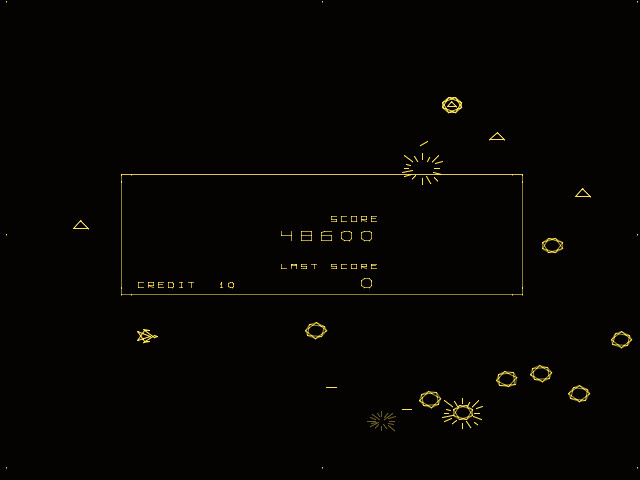Here is a detailed and descriptive caption for the image:

"A screenshot from a classic video game features a black background filled with various circular shapes that resemble alien figures. These alien-like forms appear to be the primary targets in the game. Several spacecraft are positioned strategically, seemingly engaged in combat as they fire lines resembling bullets towards the alien circles. In the center of the screen, there is a rectangular score display which reads 'SCORE: 48,600.' Below it, the display also shows 'LAST SCORE,' 'CREDIT: 10,' and '0,' indicating the player's current score and remaining credits. The vivid simplicity of the graphics epitomizes the style of retro arcade games."